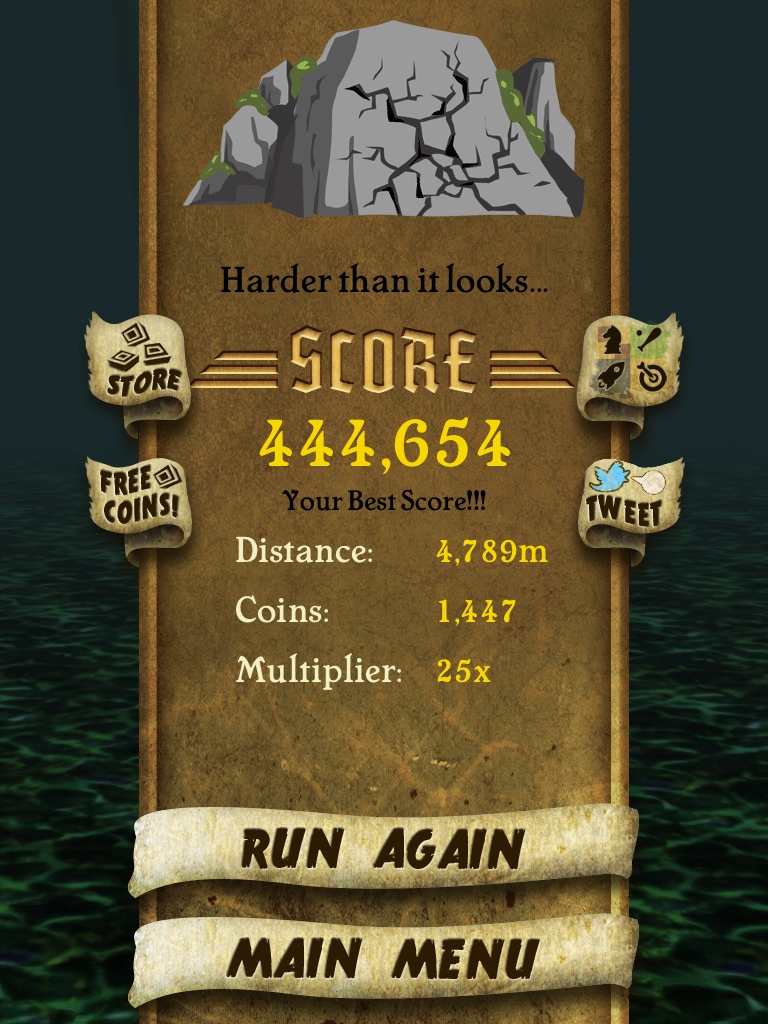This is an end-of-level screen from an arcade-style mobile game. The background features a rippling, wavy pattern in green and blue hues. At the top, a cracked gray stone boulder sits prominently, symbolizing a significant game event. Beneath the boulder, in black text, is the caption "Harder Than It Looks." A large tan rectangle in the center serves as the backdrop for the game statistics. Displayed in bold yellow text, the score reads "444,654," highlighted by "Your Best Score" underneath. Additional stats are listed below, including "Distance: 4,789 meters," "Coins: 1,447," and a "Multiplier: 25x." Two large buttons at the bottom offer the options "Run Again" and "Main Menu." On the left side, there are clickable icons labeled "Store" and "Free Coins." To the right, there are icons for social features and a "Tweet" button with a blue bird symbol. The overall aesthetic combines elements of stone, wood, and animated nature, enhancing the immersive gaming experience.